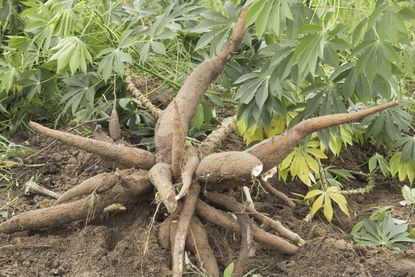The photograph, taken outdoors during the day, features a peculiar plant with a prominently exposed, large root-like bulbous structure that has seemingly been recently unearthed from the loose brown soil. The plant’s roots are thick and knotted, resembling a cluster of fat roots tied together, with limbs that taper out into thin points and show no discernible leaves. The central subject, these distinctive brown roots, occupies the middle of the image. Surrounding the main plant, the disturbed earth and scattered green weeds add to the scene's natural disorder. The background is filled with an assortment of different leaves from various trees, some star-shaped with seven petals, displaying a gradient from uniform bright green at the tops to yellow at the bottoms.